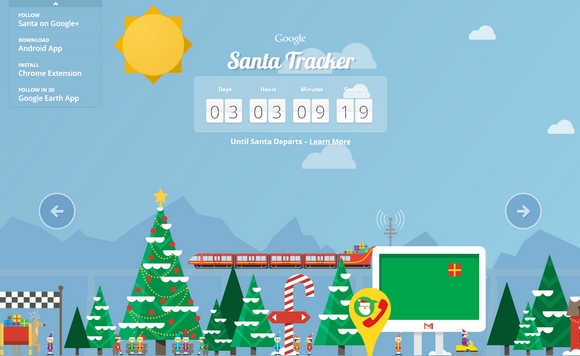The screenshot captures a festive scene from the Google Santa Tracker screensaver. Dominating the top left corner is a dropdown menu offering various options: "Follow Santa on Google Plus," "Download Android App," "Install Chrome Extension," and "Follow in Google Earth Map." The center of the image prominently displays the "Google Santa Tracker" header paired with a real-time countdown clock showing days, hours, minutes, and seconds remaining. The backdrop is a serene, blue sky dotted with fluffy white clouds and featuring a charming, cartoonish yellow sun. 

In the distance, rolling mountains add depth to the landscape. The foreground is bustling with holiday cheer—at the bottom, numerous presents scatter around, accompanied by a whimsical assortment of at least 10 tiny elves. These playful figures are interspersed between small, differently sized Christmas trees, some adorned with snow and a couple decorated with ornaments.

Additional elements further enrich the scene: a striking candy cane, a computer, and an upside-down teardrop icon depicting Santa next to a telephone. On the left side, a black and white checkered finish line stands tall next to a reindeer and Santa's sleigh. This vibrant and lively illustration perfectly encapsulates the joyous spirit of the holiday season.